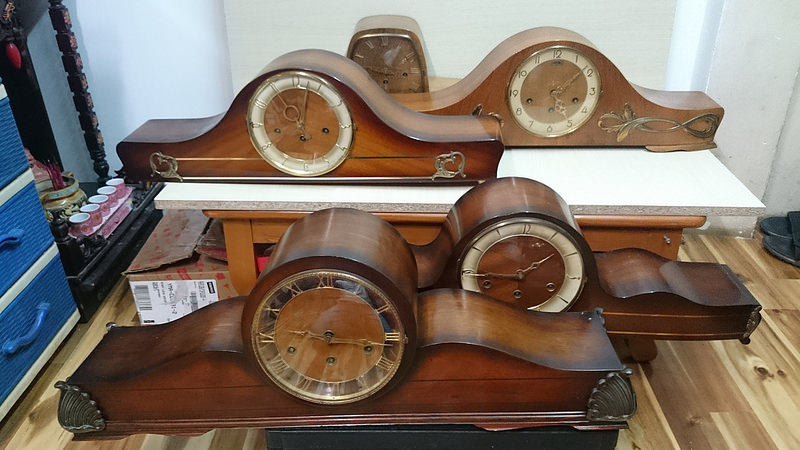This image depicts a collection of five antique-style mantel clocks arranged in a staggered line on a medium-tan wooden table. Three of the clocks feature darker cherry wood casings, while the remaining two have lighter wooden finishes—one specifically having a medium shade with a square top. The clocks are round-faced with gold decorative elements and trim. Two clocks display Roman numerals, with another two showing standard Western numerals from 1 to 12, and one has only the quadrant numbers (12, 3, 6, 9). 

Behind the clocks, additional items hint at an antique or thrift store setting: a blue and white set of tiered canvas drawers, a cardboard box with a mailing label, and miscellaneous knickknacks including a mirror with attached small spools of pink thread. The overall scene captures a quaint, nostalgic ambiance, enhanced by the surrounding wooden flooring and furnishings.